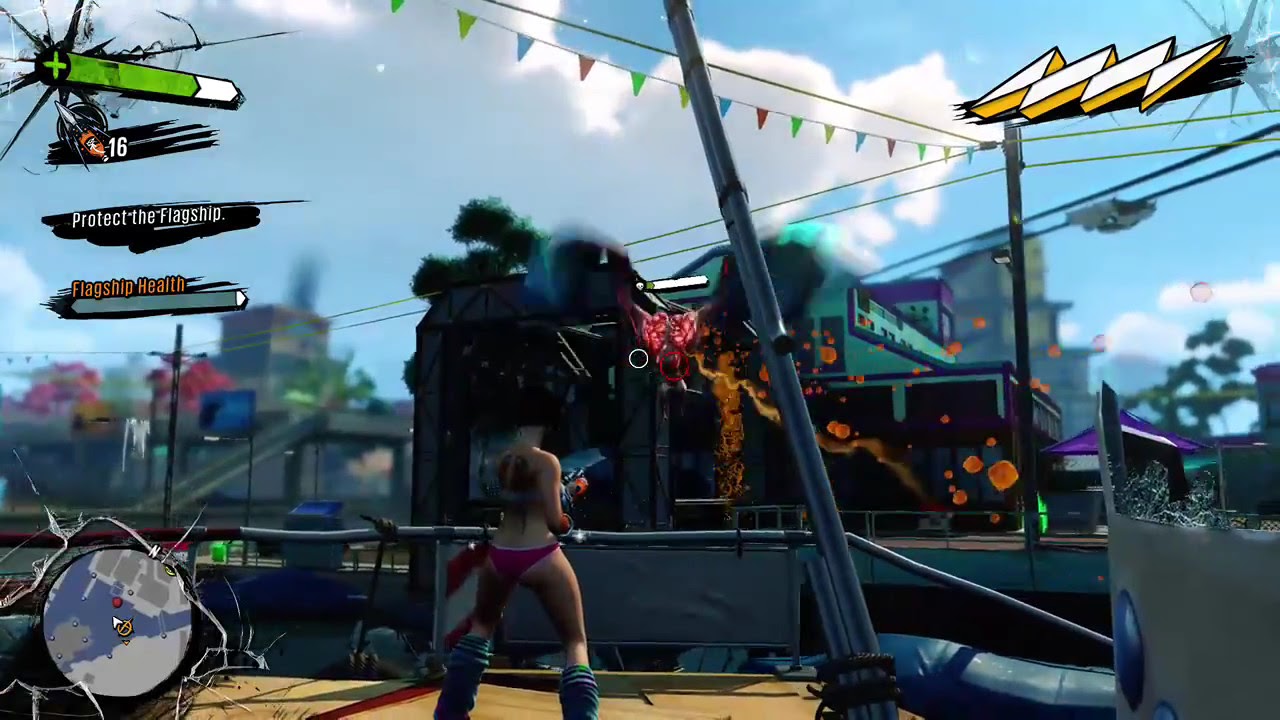The image is a high-definition screenshot from a modern video game, set in an outdoor environment reminiscent of a car sales lot due to colorful triangle banners hanging above. The scene is in broad daylight, with a clear blue sky filled with clouds. In the center of the image, a woman in a pink bikini, also wearing high socks and equipped with what appears to be Lego-like armor, is depicted aiming a machine gun. She has her back to the water and sports a tattoo on her back. Positioned on a wooden platform, possibly on the edge of a boat or a dock, she targets a burning building nearby, which appears to be on a boardwalk or dock area. The background reveals a cityscape, adding to the modern setting. The game's interface overlays include a slightly low health bar and ammo count in the top left corner, an electric energy meter in the top right, and a mini-map at the bottom left, indicating the player's location and health level. This setup suggests the game involves monster fighting in a chaotic urban environment.